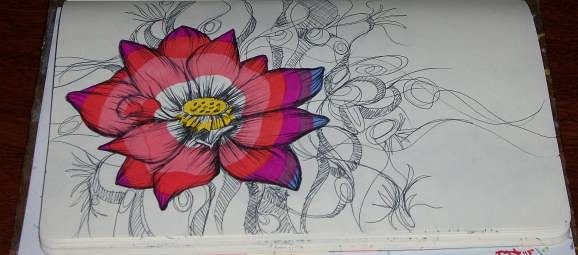This photograph captures the interior of a sketchbook, evidenced by the visible binding at the top, suggesting multiple pages. The open page features an intricate ballpoint ink drawing of a flower with flowing vines and leaves emanating from behind it. The large flower boasts multicolored petals: the right side exhibits a gradient from pink, red, and dark purple to blue at the tips, while the left side remains in shades of pink, burgundy, and dark pink. Surrounding the flower, swirling vines and floral patterns are rendered in black and white, adding contrast and depth to the artwork. The precise detailing and vivid use of color showcase the artist's skill and creativity, making this sketchbook entry truly captivating.